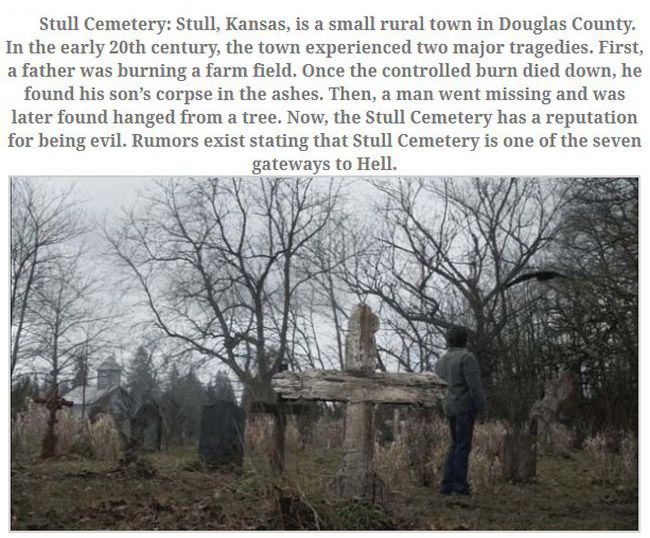This image depicts a desolate and ancient cemetery known as Stull Cemetery, located in the small rural town of Stull, Kansas, in Douglas County. The sky above is overcast with muted hues of gray, contributing to the somber atmosphere. Tall trees, stripped of their leaves, stand barren against the dreary sky, their gnarled branches reaching upward. In the foreground, the grass is brown, overgrown, and unkempt, evidencing long-term neglect. 

Dominating the center of the photo is a wooden cross, and to its right stands a solitary man, facing away from the viewer. He wears a dark jacket and pants, with dark hair, and appears to be gazing into the distance at the scattered gravestones and ancient mausoleums on the left. The scene evokes a chilling sense of abandonment and decay.

At the top of the image, text is centered, detailing the cemetery’s harrowing history: "Stull Cemetery: Stull, Kansas is a small rural town in Douglas County. In the early 20th century, the town experienced two major tragedies. First, a father was burning a farm field. Once the controlled burn died down, he found his son's corpse in the ashes. Then, a man went missing and was later found hanged from a tree. Now, Stull Cemetery has a reputation for being evil. Rumors exist stating that Stull Cemetery is one of the seven gateways to hell." The hinted-at tragedies and the cemetery's ominous lore further underscore the eerie and foreboding nature of this forgotten resting place.